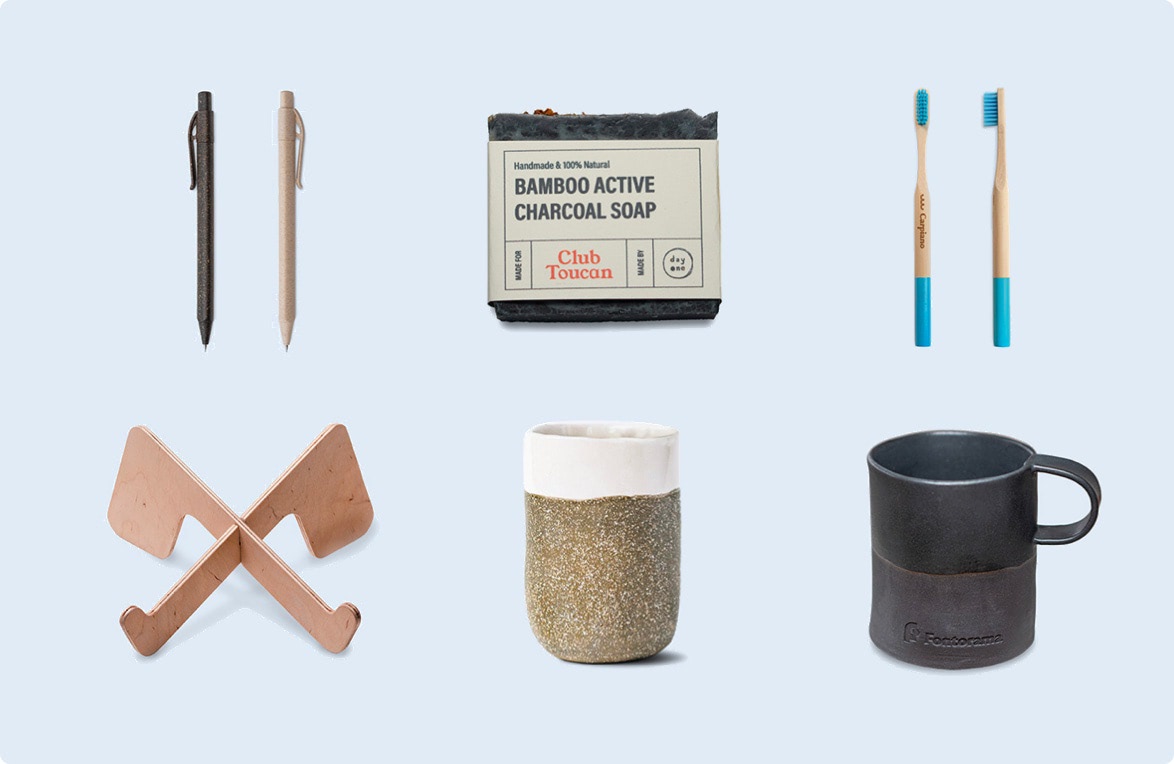The image features six distinct household items arranged on a grayish-white background in a two-row layout, each row containing three items. In the upper left corner, there are two writing instruments, one black and the other a beige-ivory color, both similar in style. At the center of the top row is a rectangular bar of black, hand-cut soap with a rustic appearance, encased in a cardboard label that reads, "Handmade 100% Natural Bamboo Activated Charcoal Soap," from the brand Club Toucan. To the right of the soap, two toothbrushes with wooden handles are positioned side by side. Each toothbrush has blue bristles and a section of blue on the handle. Located on the lower row beneath the pens, there's a distinctive black coffee cup with an unusual handle covering only half the cup's backside. Adjacent to this, a striking gold and glittery cup with a white top is placed. Finally, at the bottom left of the image, there is an intricate wooden stand with a stylized design, resembling crossed hatchets or golf clubs.